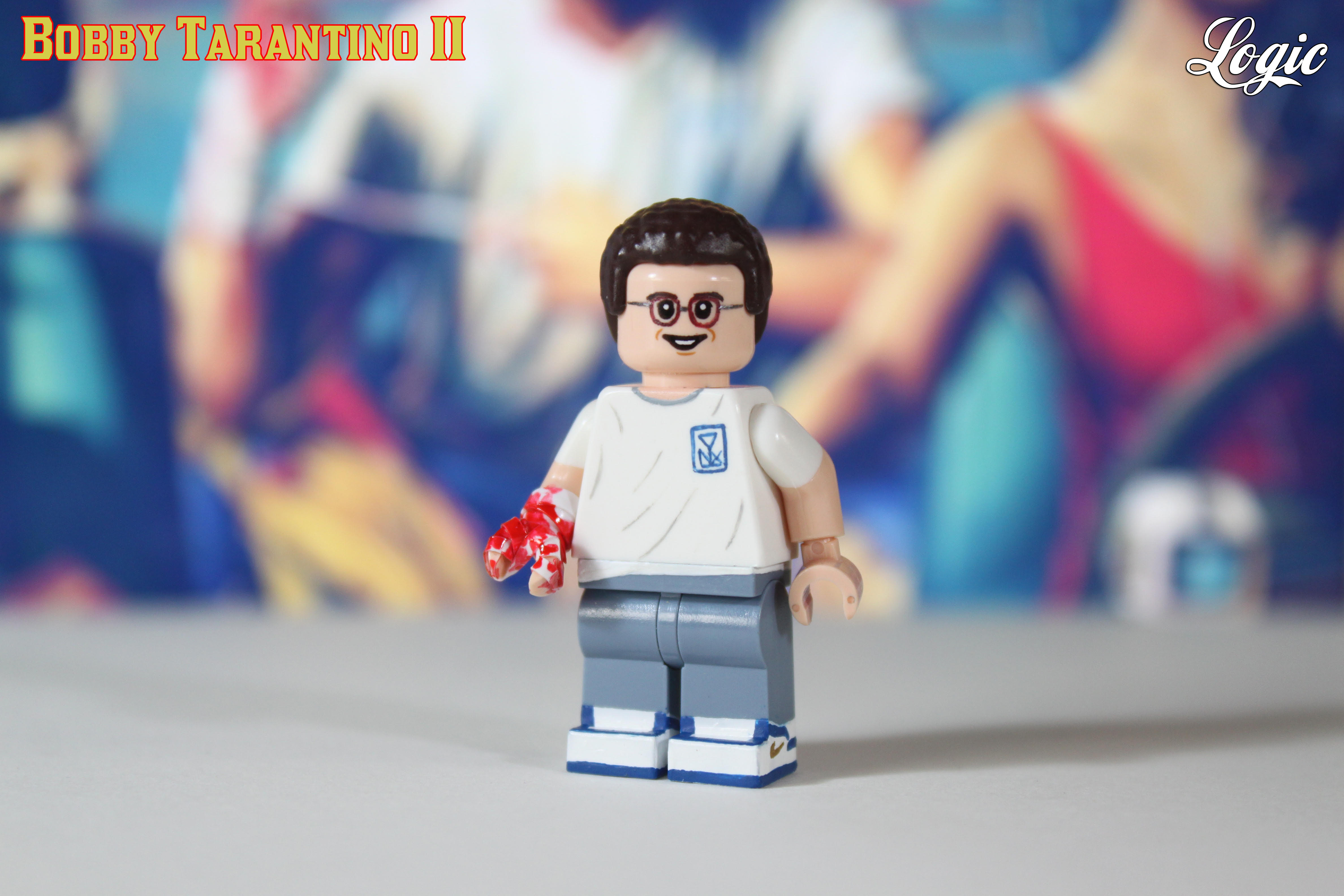The photograph showcases a detailed close-up of a Lego figure, designed to resemble a male with brown hair and glasses on a Caucasian face, smiling. The Lego man is dressed in a white short-sleeve t-shirt adorned with a blue emblem at the top right chest area, accompanied by gray pants and white and blue shoes, which possibly feature a Nike swoosh logo, though it's not distinctly visible due to the angle. Notably, the figure's right hand appears bloodied, contrasting with the normal left hand. The Lego character stands on a gray surface. Prominent text elements in the image include "Bobby Tarantino II" inscribed in a yellow, red-bordered font at the upper left corner, and "Logic" in white cursive at the upper right corner.